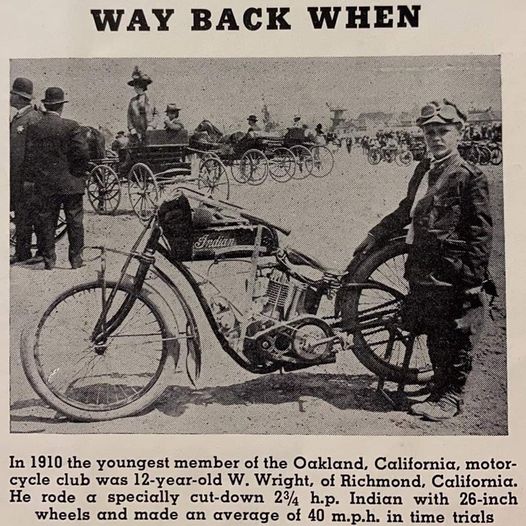The image is a black and white newspaper clipping featuring an old photograph with the caption "Way Back When" at the top and detailed text at the bottom. The photo, which looks faded and historic, shows a young boy standing next to a bicycle-like early motorcycle. The boy, who is around 12 years old, is dressed in a black jacket, loose baggy clothing, and a cap with goggles. The bottom text reveals that he is W. Wright, the youngest member of the 1910 Oakland, California Motorcycle Club, who rode a custom 2.75 HP Indian motorcycle with 26-inch wheels, achieving an average speed of 40 MPH in trials. 

In the background, there are several figures, including men in black hats and suits, as well as people sitting on horse-drawn wagons with large wheels. The scene captures an early 1900s atmosphere, highlighted by the period attire and old vehicles, which resemble early cars pre-dating the Model T.